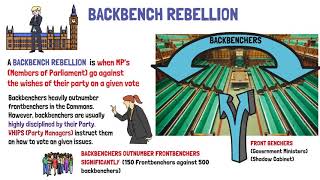The image is an informational diagram on a white background titled "Backbench Rebellion" in blue text. It explains that a backbench rebellion occurs when MPs, or Members of Parliament, vote against their party's wishes. The text, in black, red, and bluish-purple, notes that backbenchers significantly outnumber frontbenchers but are usually disciplined by party whips, who direct how they should vote. 

The left side features a person with a ponytail in a gray suit and another person with blonde hair in a gray suit standing in front of what appears to be a large building resembling those found in England. There are additional drawings that include a group of people conversing and a diagram of the parliamentary chamber. This diagram shows green rectangles representing rows of seats labeled "Backbenchers" with arrows pointing to them. The image also includes an illustration of a rebellious backbencher and another frontbencher admonishing them, alongside tiny figures to visualize the proportions of backbenchers to frontbenchers. Some of the smaller text is difficult to read.